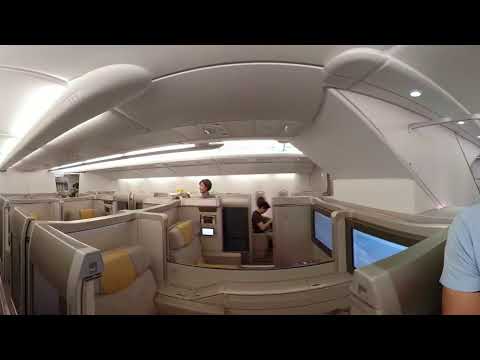In this convex, fisheye-distorted image, we see an interior setting characterized by a primarily white and light gray or beige color scheme. The scene looks like an office space with small, compact cubicles or seating areas, but it might also resemble the cabin of an airplane or a train with partitioned sections. Overhead, a white ceiling featuring circular lights can be seen, arcing in the fisheye view. To the left, more chairs are visible, and in the far background, a woman is seated in what seems to be a recliner, with another person’s head appearing behind a possible copy machine. On the right-hand side, a couple of computer monitors with light blue screens are seen, and further right, a man's shoulder and arm in a light blue shirt are partially visible, suggesting he might be the photographer. The overall setup is compact and novel, reflecting either a modern office layout or an innovative, confined airplane or train seating arrangement.